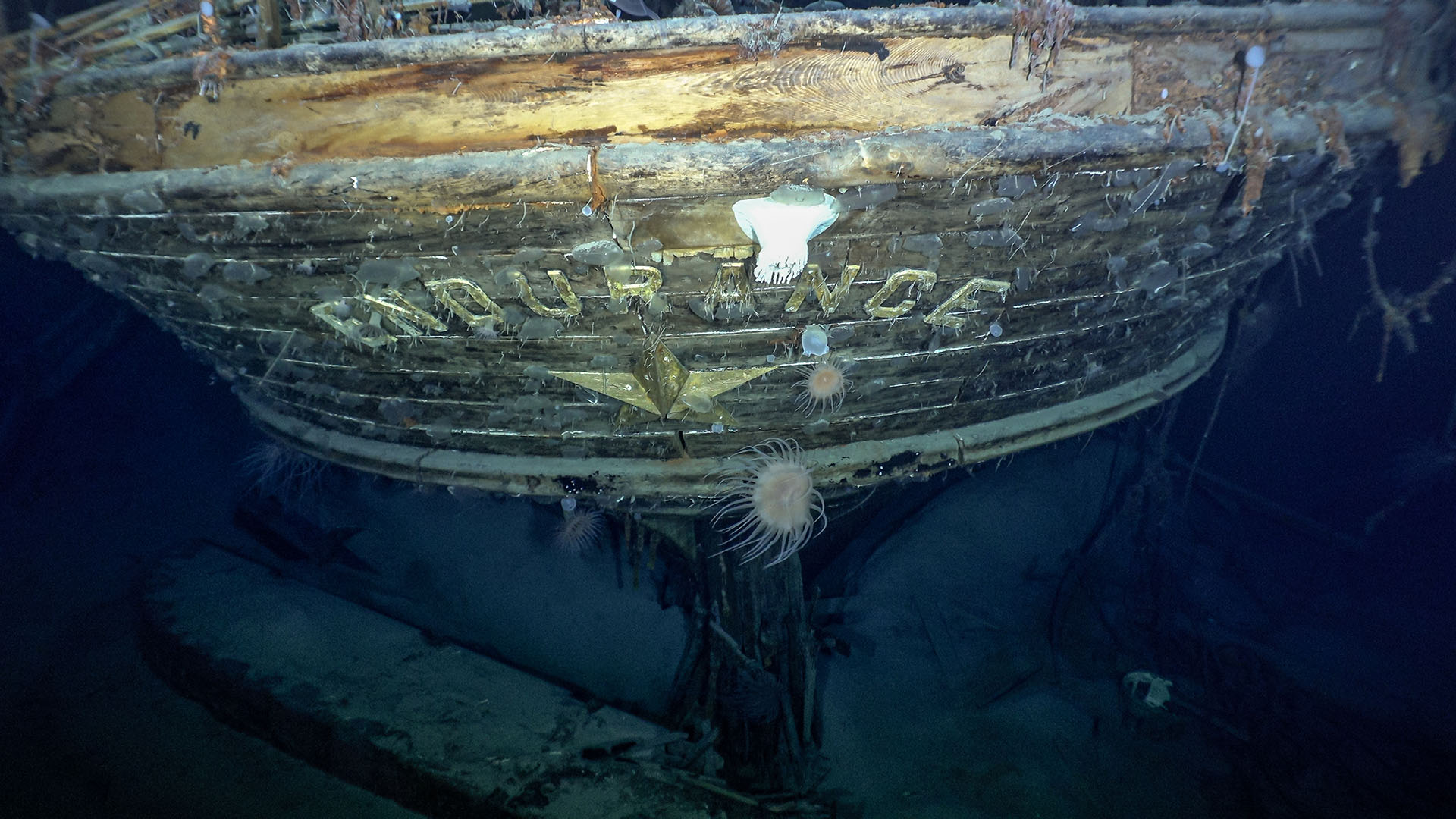The photograph depicts the bow of an old, sunken wooden ship submerged underwater, identified as the "Endurance" by the gold, uppercase letters affixed across its front. The top edge of the bow extends out of the frame, and the structure tapers to a flattened-bottom, rounded rim with a shallow, truncated cone shape. The wood appears light, weathered, and worn, showing chips and chunks, indicating prolonged exposure to the underwater environment. A white border edges the top and bottom of the bow, and a gold star emblem can be seen beneath the raised letters. The surrounding scene is dark blue, likely the ocean floor, scattered with sand, pebbles, a piece of wood to the left, and some netting-like material in the bottom right corner. In front of the bow, a small, white creature with tentacle-like extensions, resembling a jellyfish, can be seen. The image’s corners are dark, with the center illuminated, possibly by a camera flash, highlighting the shipwreck's deteriorated yet enduring state.